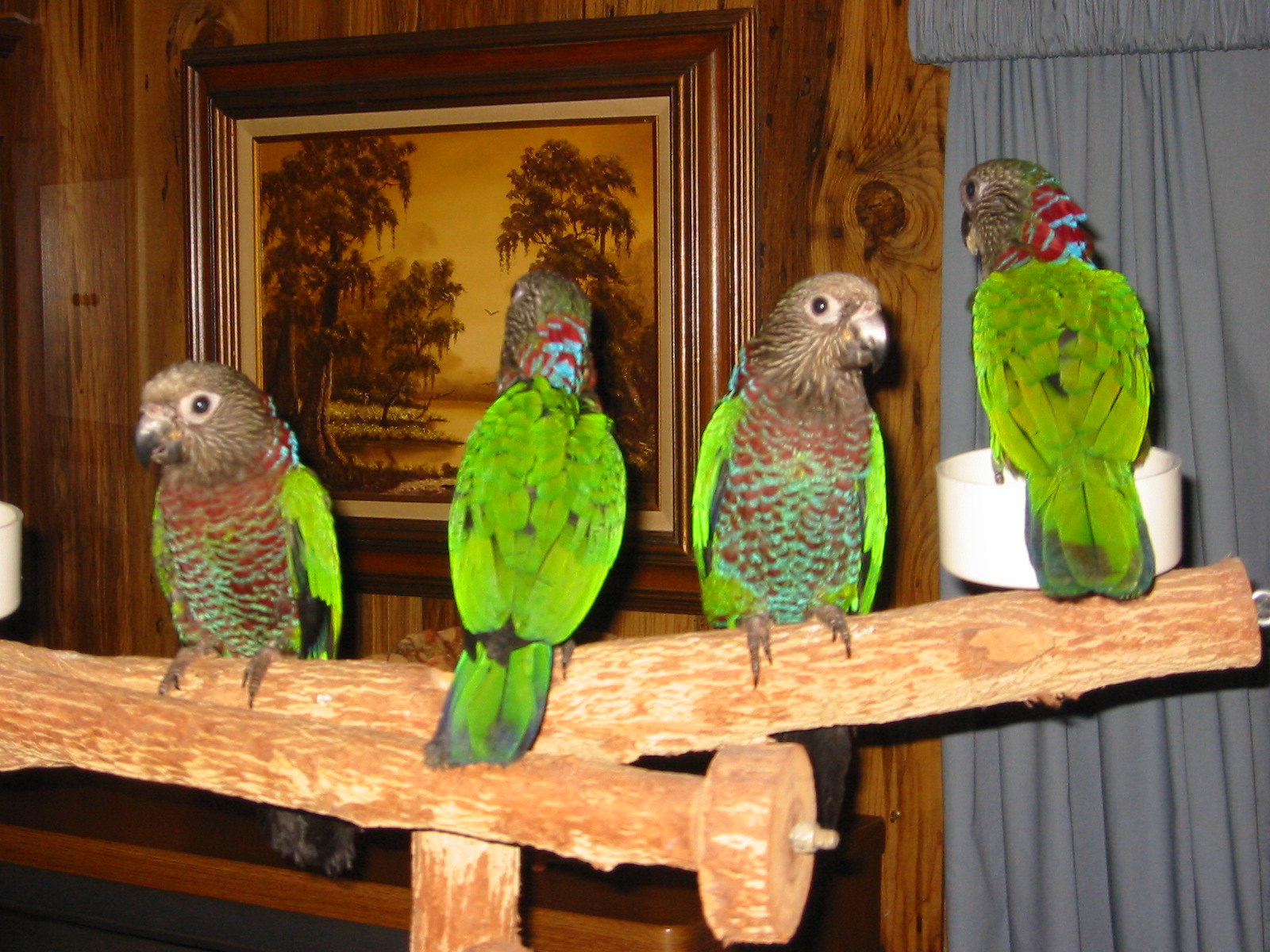In a warm, cozy living room adorned with rich, dark wooden paneling showcasing its detailed grain, we find a serene scene. On the wall, there is a beautifully framed sepia-toned landscape painting of a river meandering through a grove of trees. The painting is encased in a striking rectangular brown frame. To the right of this artwork, gray drapes cascade gracefully from ceiling to floor.

The focal point of the room, however, is an artificial wooden perch, resembling a tree branch, stationed prominently in front of the wall. Perched upon this stand are four vibrant parrots. These parrots, with their predominantly bright green plumage, are accented with splashes of red feathers on their chests and necks, and hints of brown around their faces. Their eyes, black and beady, add a lively spark to their colorful presence. Reflecting a perfectly mirrored symmetry, two of the birds face the viewer directly, while the other two face the wall, adding a unique balance to the composition. The overall ambiance of the photo captures a moment of tranquil beauty and natural elegance within the room.